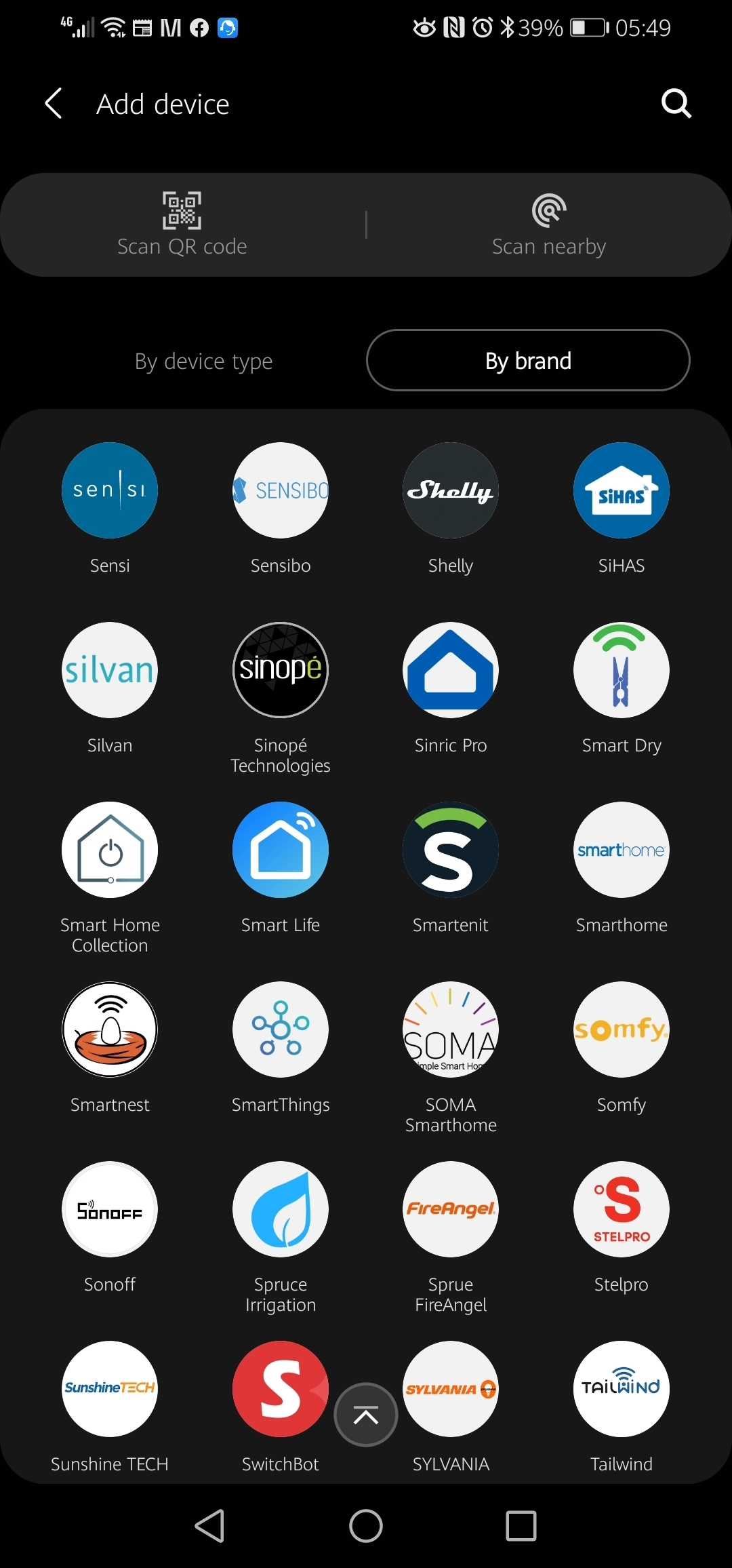This image is a screenshot taken on someone's smartphone, capturing the top menu bar and part of a home screen displaying various apps.

On the top left of the menu bar, there are several icons:
1. A 4G network indicator showing signal strength with five vertical bars, where the first three are white and the remaining two are gray.
2. A Wi-Fi signal icon.
3. A calendar or newspaper icon.
4. The letter "M" icon.
5. The Facebook icon, which is a circular icon with an "F" in the center.
6. A blue square icon featuring a cartoon person.
7. An eye icon.
8. An icon resembling a chain or an "S" enclosed in a box.
9. An alarm clock icon.
10. The Bluetooth symbol.
11. A 39% battery indicator presented as a rectangular icon filled partially in white.
12. The current time is displayed on the far right.

In the main content of the screenshot, the home page features a section titled "Add Device," accompanied by a leftward-pointing arrow. To the right of this title, there is a magnifying glass icon for search functionality.

Below this, a gray cylindrical banner presents two buttons:
1. A button with a QR code icon labeled "Scan QR Code."
2. A button with a signal icon inscribed in a circle, labeled "Scan Nearby."

Additionally, there are two tabs labeled "By Device Type" and "By Brand," with the "By Brand" tab currently selected as indicated by a border around it.

The list beneath features apps or options organized in a 4x6 grid format, totaling 24 items. These items are sorted alphabetically and each displays a circular logo above the name of the app or option. The apps listed from top to bottom are:
1. Sensi
2. Sensibo
3. Shelly
4. Siha
5. Sylvan
6. SinoPay Technology
7. Siric Pro
8. Smart Dry
9. Smart Home Collection
10. Smart Life
11. Smart Innit
12. Smart Home
13. Smart Nest
14. Smart Things
15. Soma Smart Homes
16. Home 5
17. Sound Off
18. Spruce Irrigation
19. Spruce Fire Angel
20. Stealth Pro
21. Sunshine Tech
22. SwitchBot
23. Sylvania
24. Tailwind

This detailed depiction captures the intricate layout and specific icons present in the screenshot, giving a clear understanding of the smartphone's display at that moment.